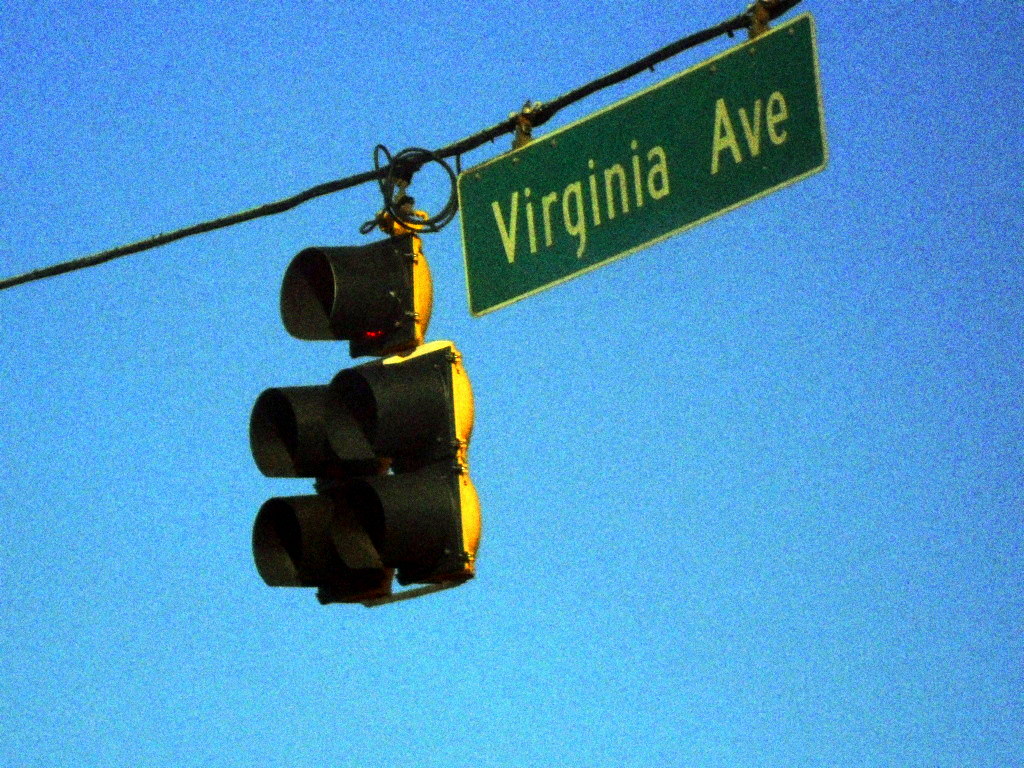The photograph captures a traffic light and street sign suspended from a power line against a vibrant blue sky, creating a striking contrast. The traffic light is predominantly black with a yellow back, and its design is unusual, featuring five segments: a top light and four clustered below. While it's typical for these lights to indicate red, yellow, green, and directional arrows, none of the lights are lit in the photo. To the right of the traffic light, a green street sign with white lettering reads "Virginia Ave." The image appears to be taken from a distance with a significant zoom, resulting in a pixelated and grainy sky. The simplicity of the composition—the blue sky, the black and yellow traffic light, and the green street sign—creates a minimalist yet evocative scene.